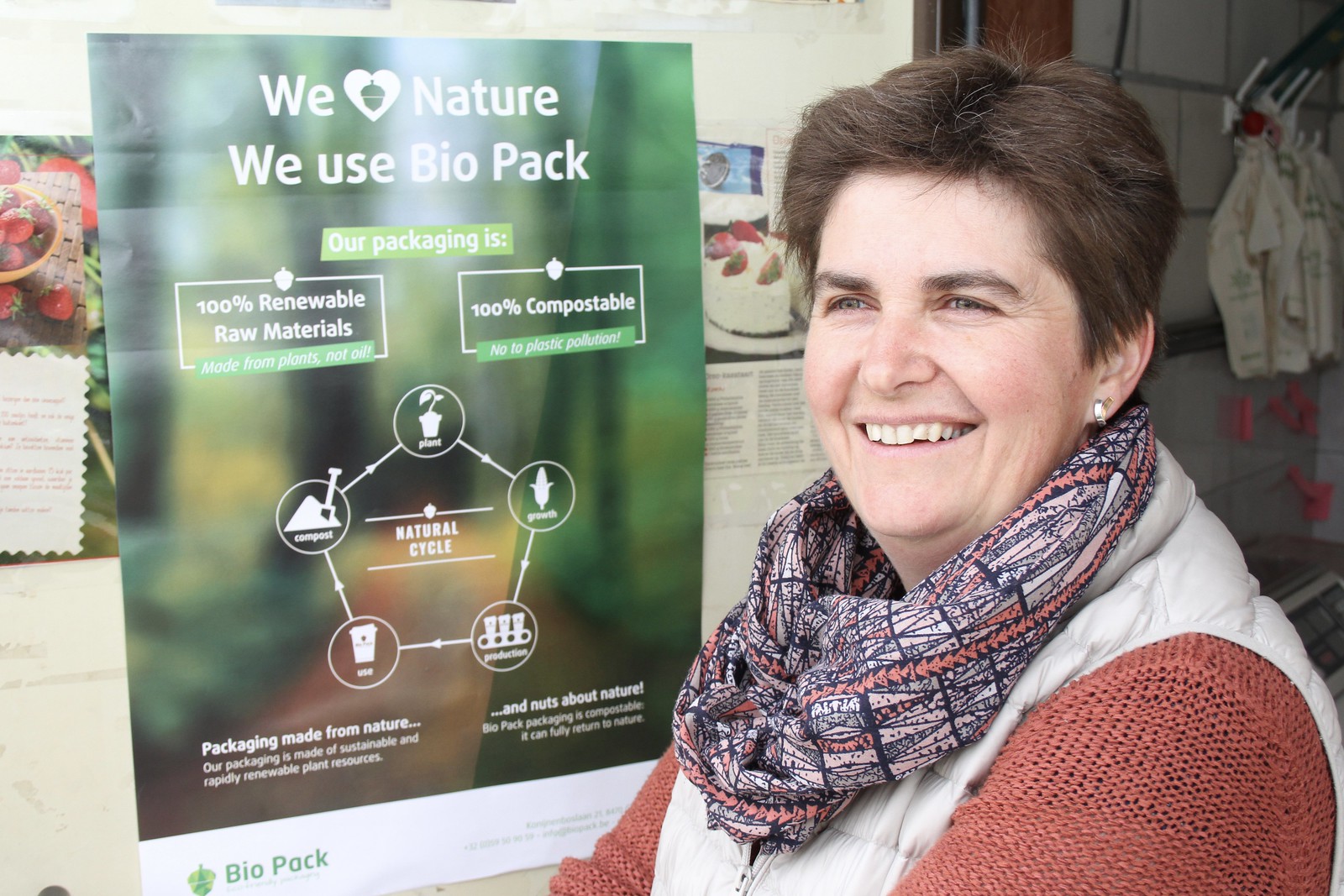In this image, a woman with short, reddish-brown hair and green eyes is posing for a picture. She is wearing a long-sleeve red sweater layered with a white vest coat, and a patterned scarf in shades of brown, red, and white wrapped around her neck. She accessorizes with white stud earrings and is captured smiling while looking off-screen to the right. Her hairstyle is medium in length, adding a touch of elegance to her appearance. To her left, there's a green sign with white text, promoting Biopack. The sign reads, "We Heart Nature. We use Biopack," followed by a graph that illustrates the company's commitment to eco-friendly packaging. The graph is topped with the phrases "100% compostable" and "100% renewable raw materials." The background includes various posters and signs, reinforcing the environmental theme. The setting appears to be a company's indoor location, suggesting it might be a business headquarters or office environment, taken during daylight hours.